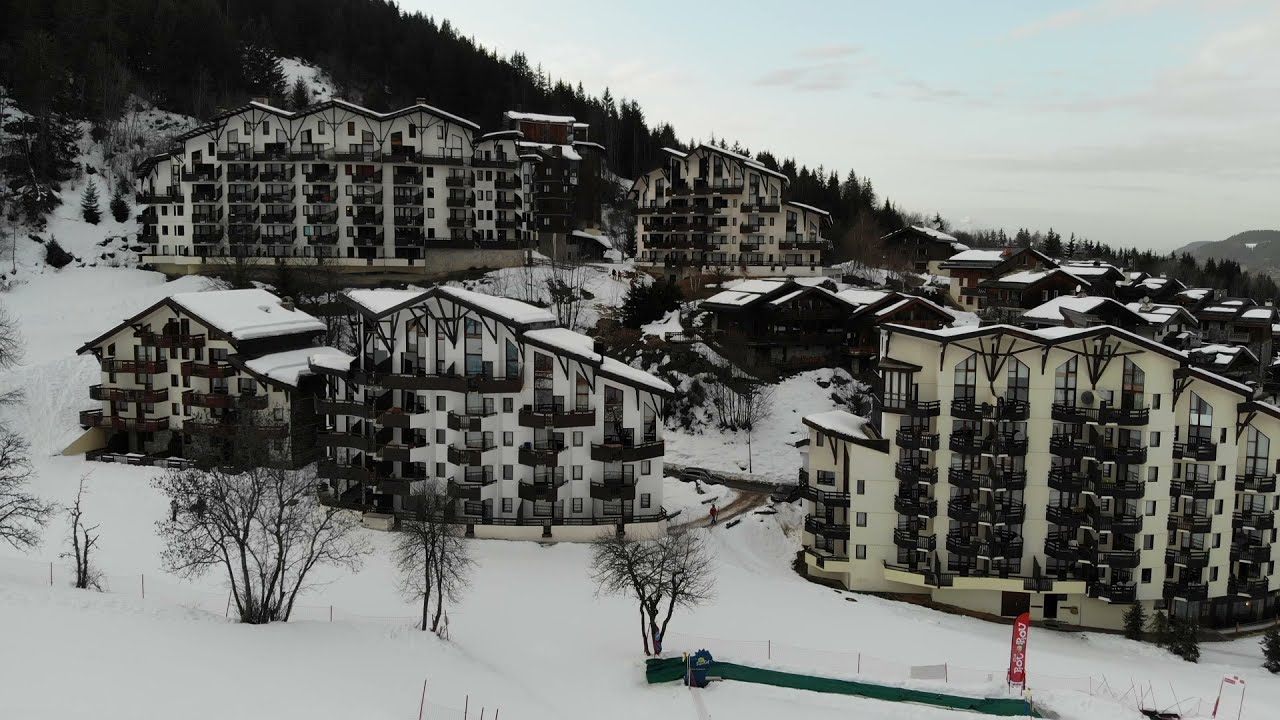This photograph captures a picturesque, snowy, daytime scene of a neighborhood nestled in a mountainous area, possibly reminiscent of Colorado or Utah. Dominating the foreground are multiple large, white and gray buildings that stand five to six stories high, each adorned with brown, slanted rooftops blanketed in snow. These buildings, likely apartment complexes or chalets, boast numerous windows and balconies, characteristic of a mountain resort or ski area. Clear, paved roads snake their way up to the buildings, contrasting with the untouched snow on the ground and rooftops. Sparse, leafless trees stand before the structures, adding to the wintry ambiance. In the background, a large hill or mountain peaks, covered with dark, towering pine trees, framing the snowy resort-like scene.